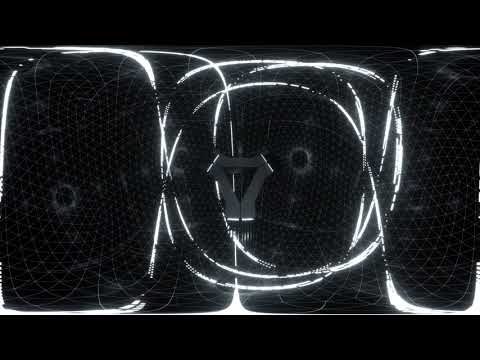The image features a dark, black background resembling black netting or a grid commonly seen in physics illustrations. At the center of the photo, there's a silver metallic emblem shaped like a smoothed-down triangle, with its main point pointing downwards. Inside this emblem is a smaller, more traditionally shaped triangle cut-out. Flanking this central symbol are white lines, including a few larger, not entirely symmetrical forms. To the left and right, there are vertically aligned rectangular lines. Some of these lines form circles, arcs, and rhombus shapes, which crisscross and intersect, creating an intricate white grid over the black background. The white lines have a textured, hand-drawn appearance with breaks, indicating they might be sketched or painted. This detailed confluence of shapes and lines suggests an abstract piece of artwork or a still image from a video screen depicting a stylized representation of space and time.